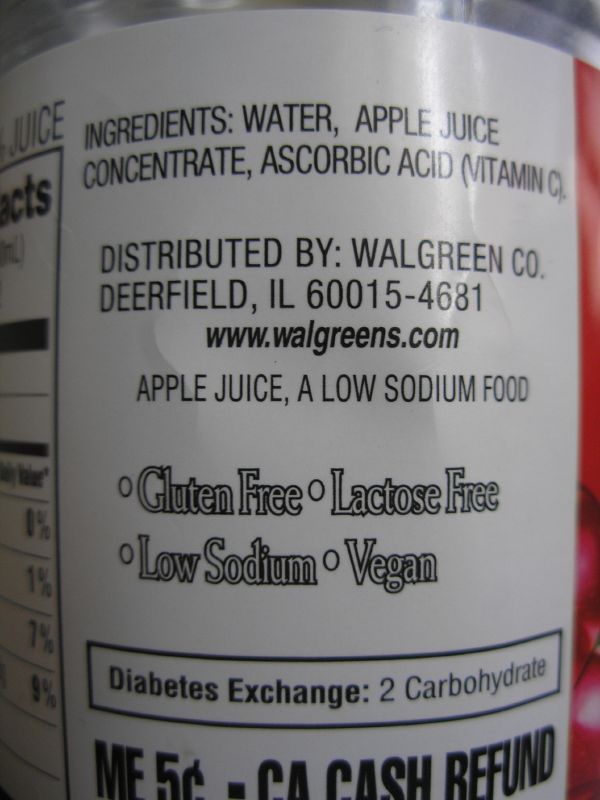This image features a close-up of a label on a bottle, presumably of apple juice, as indicated by the repeated mention of apple juice concentrate among the ingredients listed. The label itself is predominantly white with red edges and black writing. Highlighted on the label are the ingredients: water, apple juice concentrate, and ascorbic acid (vitamin C). It states that the product is distributed by Walgreens Co., headquartered in Deerfield, Illinois, 60015-4681, and provides the website www.Walgreens.com. Additionally, the label emphasizes key dietary features in bold or with bullet points: gluten-free, lactose-free, low-sodium, and vegan. There's also a box mentioning diabetes exchange with two carbohydrates. Other notable details include ME 5 cents with a reference to California cash refund. The partial nutrition facts visible show percentages of 0%, 1%, 7%, and 9%. The overall composition suggests an emphasis on health-conscious and dietary-specific attributes in an apple juice product, likely a Walgreens brand, with the visual framing including a glimpse of both nutritional information and a small red logo that might depict apples.